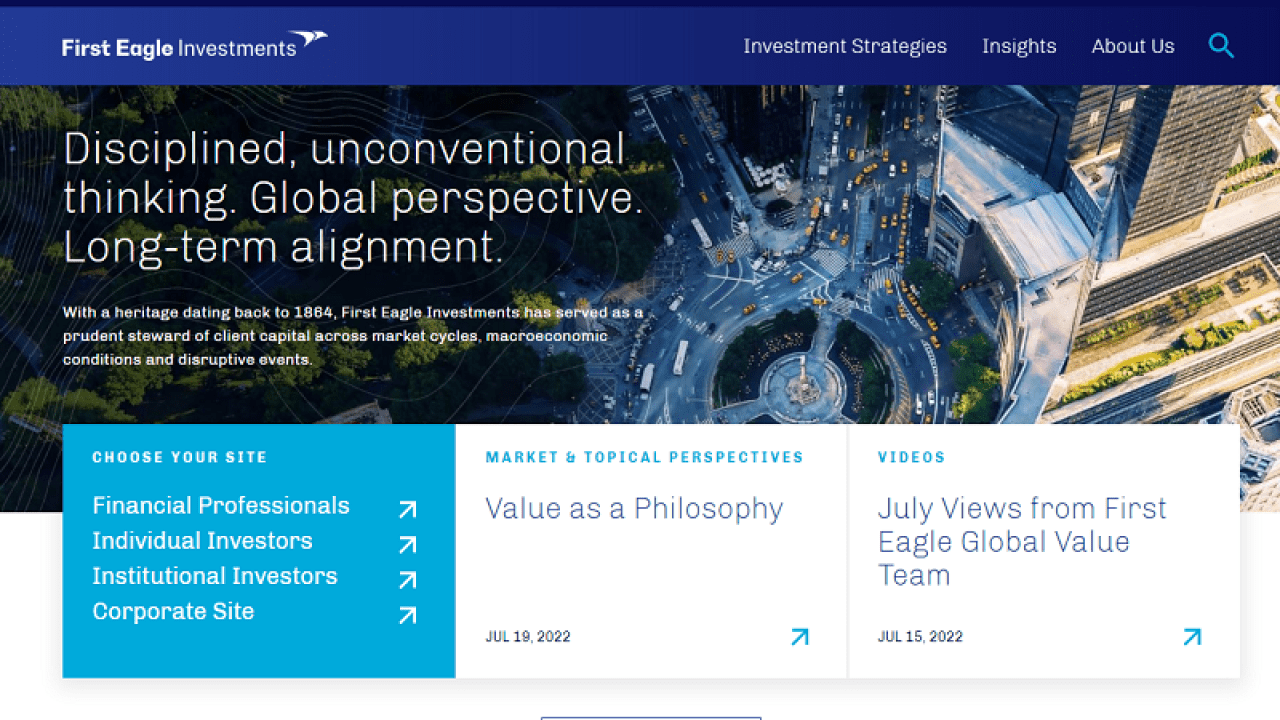The website interface for First Eagle Investments features a prominent blue navigation bar across the top. On the right-hand side of the blue bar are white text columns labeled "Investment Strategies," "Insights," and "About Us." Dominating the center of the page is a high-angle image of a cityscape showcasing a bustling street below, encircled by a roundabout, flanked by high-rise buildings on the right, and a garden area.

To the left of the garden, there is a dark green treed area with white text overlaying it that emphasizes the company's principles: "Disciplined, Unconventional Thinking, Global Perspective, Long-Term Alignment." Just below this, a tagline contextualizes the company’s legacy: "With a heritage dating back to 1864, First Eagle Investments has served as a prudent steward of client capital across market cycles, macroeconomic conditions, and disruptive events."

Beneath this text is a functional bar highlighted by a blue square prompting users to "Choose Your Site." The options listed include "Financial Professionals," "Individual Investors," "Institutional Investors," and "Corporate Site." In the central part of the webpage, a highlighted box presents a featured insight titled "Market and Topical Perspectives: Value as a Philosophy," dated July 19, 2022. 

To the left, another box promotes video content titled, "July Views from First Eagle Global Value Team," dated July 15, 2022. This visual arrangement delivers a streamlined yet detailed overview of the website’s focal points, reflecting First Eagle Investments' deep-rooted expertise and broad market insights.